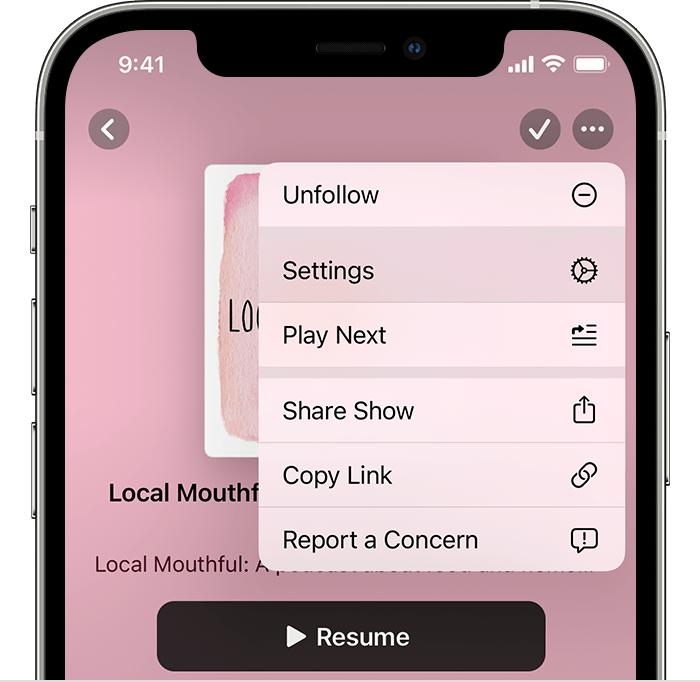This image is a detailed screenshot showcasing a mobile phone interface, likely captured during an app demonstration. Prominently on the right side is a vertical dialogue box with a series of action items. At the top of this box, in clear bold text, it reads "Unfollow," immediately followed by "Settings" underneath it. The subsequent item listed is "Play Next." A noticeable gray separator bar divides these initial options from the subsequent items. Below the separator, the list continues with "Share," followed by "Show," "Copy Link," and finally "Report a Concern." Each action item is accompanied by a corresponding icon for easy identification. For example, the "Copy Link" option is illustrated with an icon depicting two interlinked chain links, symbolizing the action of copying a link. The interface details and orderly structure suggest user-friendly navigation elements typical of modern mobile applications.